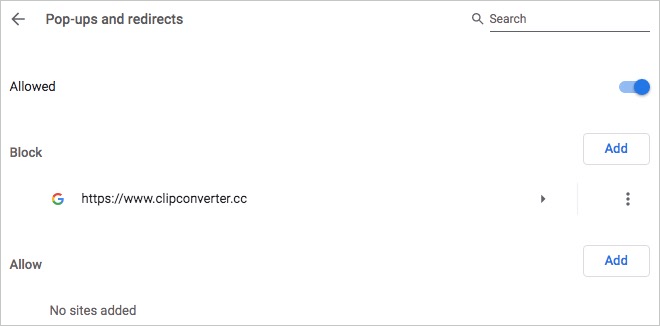This is a screenshot of a settings menu on a phone or tablet designed for managing website permissions. The menu has a predominantly black and white color scheme, with blue buttons here and there. At the top-left corner, there's a back button, and on the upper-right corner, there are a search icon and a contacts icon. 

The central part of the screen shows options for managing pop-ups, blocked sites, and allowed sites. Permissions are divided into "Block," with one entry for "https://www.clipconverter.cc" displayed alongside a Google insignia, indicating it has been blocked. Below this, there are "Add" buttons next to both "Block" and "Allow" sections, allowing users to add more sites to either list. Additionally, there's an "Allow" section for pop-ups, which currently shows "No sites added." 

Navigation within this settings menu appears to involve an arrow or a three-dot drop-down menu next to blocked entries, providing further customization options. Overall, the interface is clean and straightforward, with intuitive controls for managing website permissions.